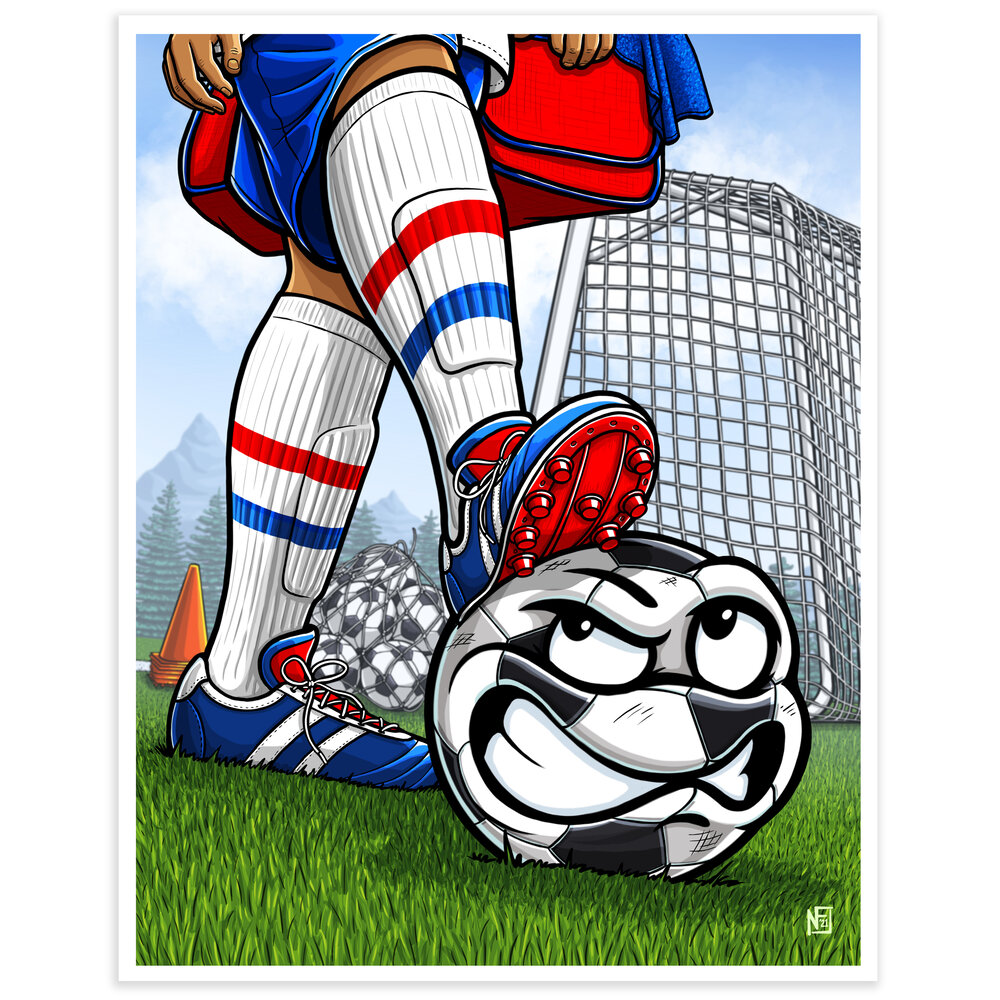The illustration showcases a stylized, cartoon drawing of a soccer player, whose body is cut off just above the knees, leaving only their legs and the ends of their hands visible. The player is dressed in a red, white, and blue outfit, featuring blue shorts, a white jersey, and knee-length white socks with red and blue stripes crisscrossing over their shin guards. Their right leg is propped on top of a gray and white cartoon soccer ball with a humanized, grimacing face that looks back up at the player, almost growling. Their left foot is grounded behind the ball. The player wears blue cleats with red bottoms, prominently displayed as the right shoe rests on the expressive soccer ball. Accompanying the player is a red sports bag slung behind their legs.

In the background, to the left, there is a stack of orange cones, and towards the center, a bag filled with soccer balls sits between the player's feet. On the right, the background features a soccer goal. The scene is set against a grassy field, and further back, to the left, are trees and mountains, while on the right looms the outline of a large building. The playful yet detailed illustration captures a humorous and dynamic moment in the world of soccer, emphasizing the clash between the human and the animated ball.